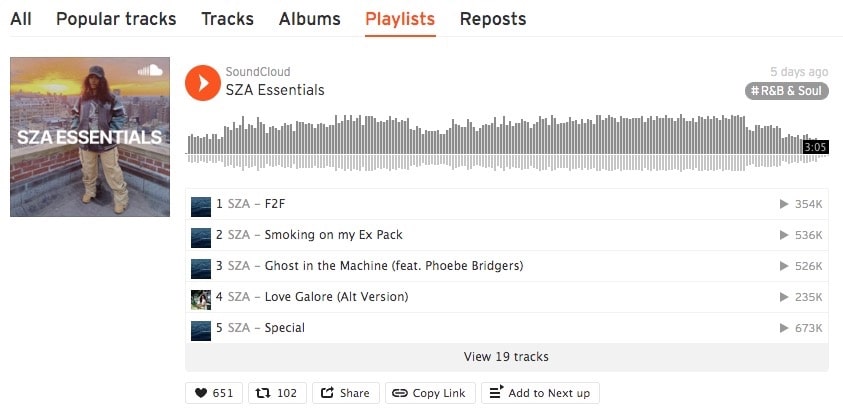This image is a detailed screenshot of the SoundCloud music program interface. At the top left corner, the SoundCloud logo is visible against a white top banner that features menu options reading: "All," "Popular Tracks," "Tracks," "Albums," "Playlists," and "Reposts." The "Playlists" option is highlighted in red and underlined.

Central to the display is a highlighted playlist titled "SZA Essentials," featuring an album cover with an image of a woman wearing a hat, standing on a rooftop with a cityscape and a setting sun in the background. This album cover is set within a square frame. 

The main section of the display shows music playback details. A black button on the right side of a progress bar indicates the track length of three minutes and five seconds. An orange circle with a white right arrow serves as the play button. Below this, a list of songs in the playlist is shown, including "F2F," "Smoking on My Ex-Pack," "Ghost in the Machine" featuring Phoebe Bridgers, "Love Galore (Alt Version)," and "Special."

Beneath the playlist, there is a thin gray button labeled "View 19 Tracks," hinting at more songs within the playlist. A row of interaction buttons follows, indicating "651" likes marked by a heart, "102" shares, alongside buttons for sharing, copying the link, and adding to "Next Up."